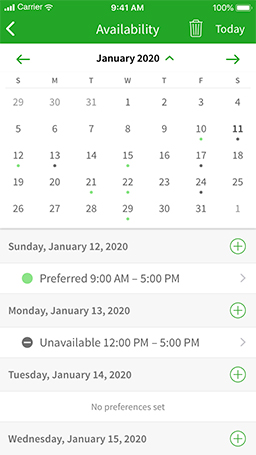Screenshot depicting a mobile phone screen showing a calendar interface. The top of the screen indicates the time as 9:41 AM with full battery availability at 100%. The current date highlighted is "January 2020," and navigation arrows on either side allow switching between months.

The calendar grid displays the days of the week from Sunday (S) to Saturday (S). The date range shows the end of December 2019 with the numbers 29, 30, and 31 shaded, indicating they belong to the previous month. January 2020 is presented with dates from 1 through 31, while the first day of February is shaded, marking the transition to the next month.

Below the calendar grid are detailed appointments and availability statuses:
- Sunday, January 12, 2020: Available from 9:00 AM to 5:00 PM.
- Monday, January 13, 2020: Unavailable from 12:00 PM to 5:00 PM.
- Tuesday, January 14, 2020: No preferences set.
- Wednesday, January 15, 2020: Status unspecified.

Each date entry is accompanied by a green circle with a plus sign, likely indicating the option to add or edit events.